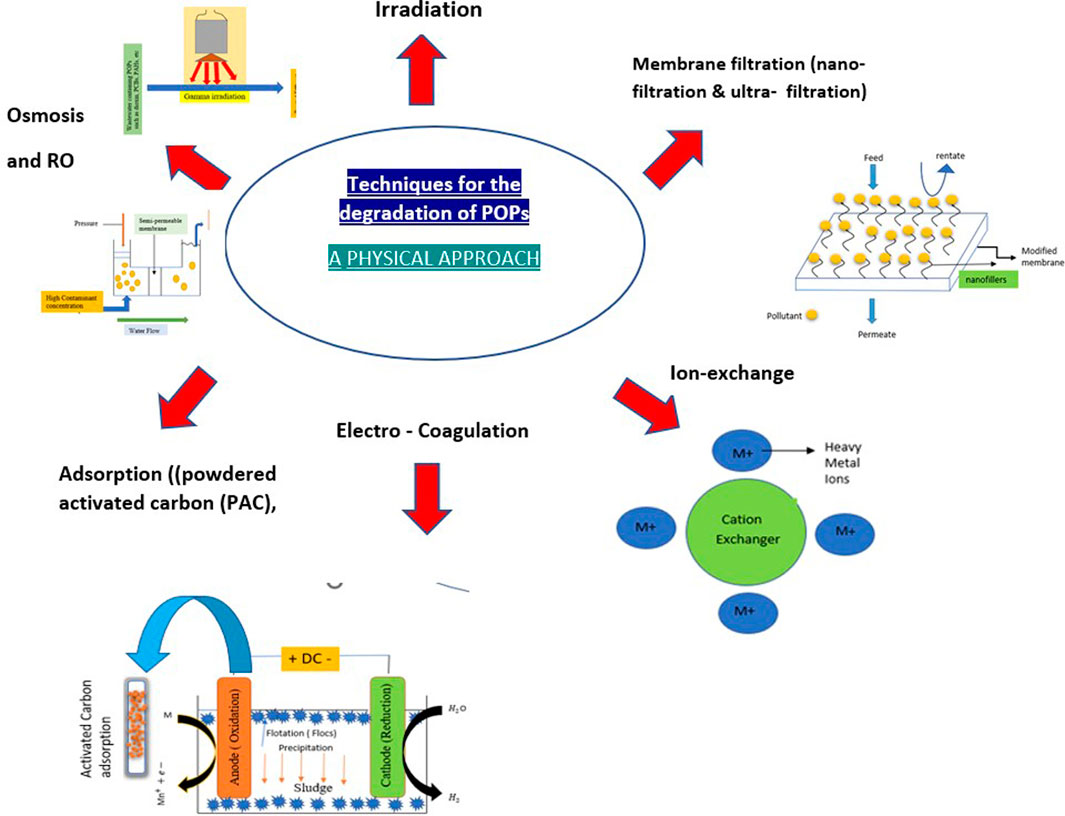In the image, a prominently large poster is displayed with the word "Irradiation" boldly printed at the top. Below this title, a red arrow points upwards, indicating irradiation as a key topic. Dominating the center of the poster is a sizable, blue oval shape with a white interior that reads "Techniques for the Degradation of POPs: Physical Approach." The oval is designed with blue and green hues.

To the right, a series of red arrows branch out, each pointing toward different methods listed on the poster. One arrow directs attention to "Membrane Filtration," which is further specified into "Nano Filtration" and "Ultra Filtration." Another red arrow points towards "Ion Exchange," specifying the use of a "Cation Exchanger" for removing "Heavy Metal Ions." 

Continuing downward, more red arrows highlight "Electrocoagulation," "Adsorption" (with a note of "Pallid Activated Carbon"), and finally "Osmosis and RO" (Reverse Osmosis). At the bottom of the poster, the process concludes with another red arrow indicating "Activated Carbon Adsorption." Each segment is meticulously illustrated with connecting arrows to demonstrate the flow and relationship among these physical approaches to degrading POPs (Persistent Organic Pollutants).